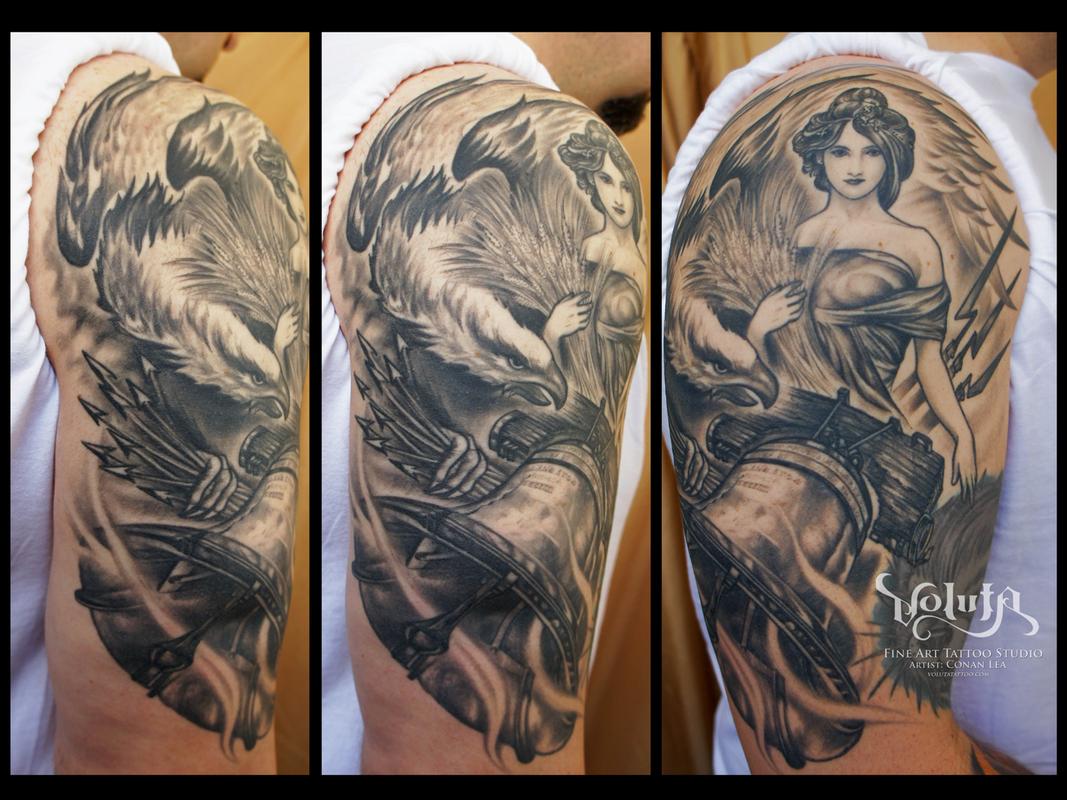The image showcases a detailed tattoo from three different angles on a man's upper arm, arranged side-by-side with black spaces in between, all framed in black. 

- **Leftmost Photograph:** Taken from the back side of the arm, revealing part of the man’s white rolled-up sleeve and white boots. This view captures the back and side of the tattoo, highlighting arrows, wing-like structures, and a part of an eagle's head. The background is predominantly brown.

- **Middle Photograph:** Provides a more frontal view of the tattoo, depicting a woman in a strapless dress, holding a bundle of wheat. The design also includes an eagle and a bell at the bottom. 

- **Rightmost Photograph:** Offers a straight-on perspective of the tattoo, where the woman’s full figure is visible along with part of the bell. The eagle is partially hidden, and there are lightning bolts to the woman's right. 

The tattoo follows an American theme, featuring a beautiful woman (possibly an angel), an eagle, and a bell, with fine detailing in black ink. At the bottom-right corner of the image is the text "Voluta Fine Art Tattoo Studio" along with the artist's name, Kunan Lee, and the website address, volutatattoo.com.